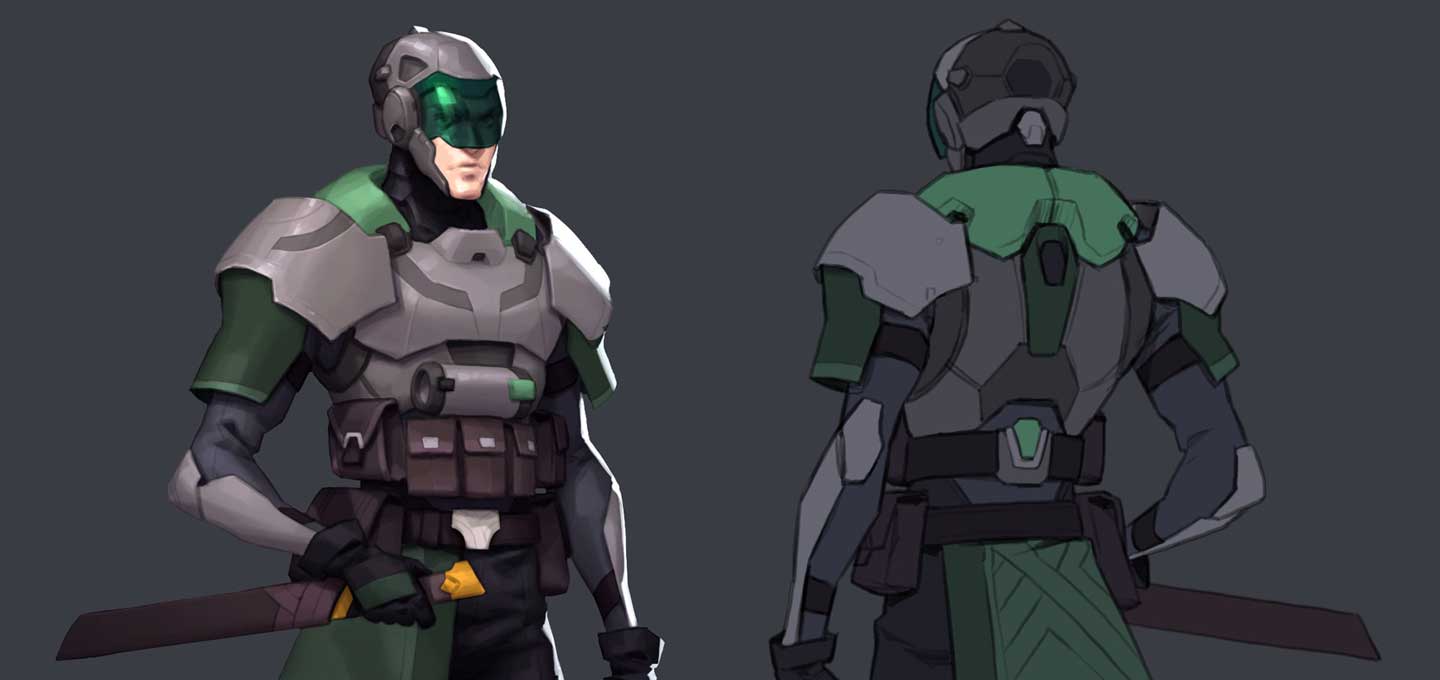The horizontally aligned rectangular digital artwork depicts a character wearing futuristic armor. The character appears twice in the same image: facing forward on the left side and with its back to the viewer on the right side. This superhero-like figure's armor features a blend of green and gray colors. The front-facing character wears a gray helmet with a green visor covering the eyes, leaving only the nose, mouth, and chin visible. The armor includes a green and gray chest plate, armbands, and green sleeves. The character’s right hand grips a gray sword, accented with yellow parts, sheathed at the hip. Black gloves are visible on both figures, and a green back skirt is noted on the rear-view character. Positioned around the character's waist is a belt with several pouches, including two larger ones on either side. The background of the image is a solid dark gray, emphasizing the detailed design and posture of the two armored figures.